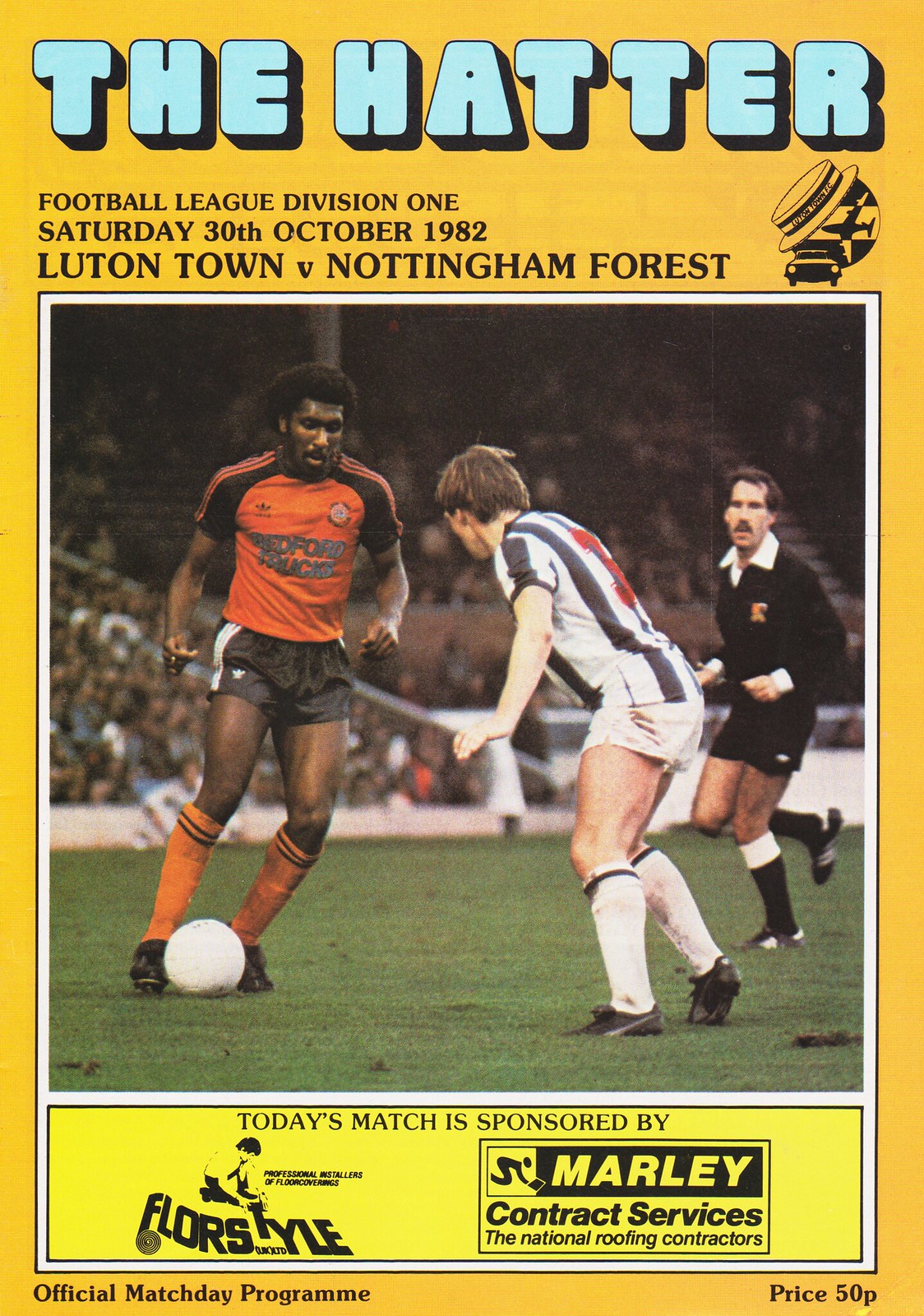The vibrant cover of the soccer magazine features a deep yellow background without any border. Dominating the top in large, bold light blue bubble letters with black shadows is the title, "THE HATTER." Directly beneath it, in all capital black letters, it reads: "FOOTBALL LEAGUE DIVISION 1 SATURDAY 30TH OCTOBER 1982 LUTON TOWN V NOTTINGHAM FOREST." The central focus of the cover is a large, colorful photograph capturing a dynamic moment during a soccer match. 

In the foreground on the left, a black man with a short afro, dressed in an orange shirt with black sleeves, thin black shorts, and long knee-high orange socks, skillfully controls the ball on a green field. Opposing him is a white man with short brown hair, wearing a white jersey with black stripes, black shorts, and socks, actively defending and attempting to intercept the ball. In the background, a white man with a mustache clad in a black uniform with a white collar appears to be officiating the match. The photograph is set against what seems to be the field with stands full of spectators, adding to the ambiance of the scene.

At the bottom of the cover, a yellow banner announces the sponsorship in black text: "Today's Match is sponsored by Flores Flyle and Marley Contract Services." Additionally, it states, "Official Match Day Program, price 50p," indicating the magazine's purpose and cost.